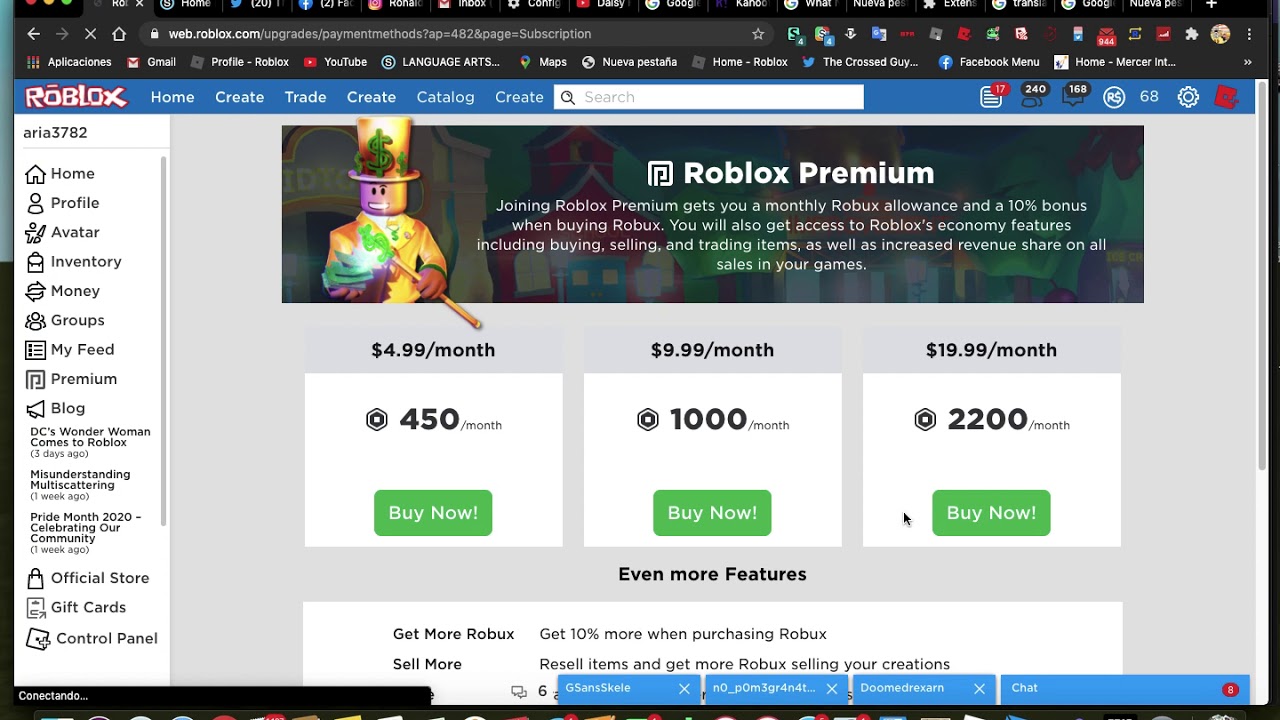The image displays a computer screen with the URL "www.roblox.com/upgrades/payment" entered in the search bar. At the top of the screen, multiple tabs are visible, including "Roblox Home," "Create," "Trade," "Catalog," and "Create" repeated thrice, along with a search bar. The user has 17 messages, 240 friends, 168 notifications, and has their username next to the number 68. There is also a settings menu icon.

Beneath these tabs, a section titled "Roblox Premium" describes the benefits of joining the service. It mentions that membership includes a monthly amount of Robux, a 10% discount on Robux purchases, and access to various Roblox economy features such as buying, selling, and trading items, along with increased revenue share on all sales in your games. The membership options are listed as $4.99/month for 450 Robux, $9.99/month for 1000 Robux, and $19.99/month for 2200 Robux, each with a "Buy Now" button next to them. On the left side of the screen, there are additional sections of the site highlighted.